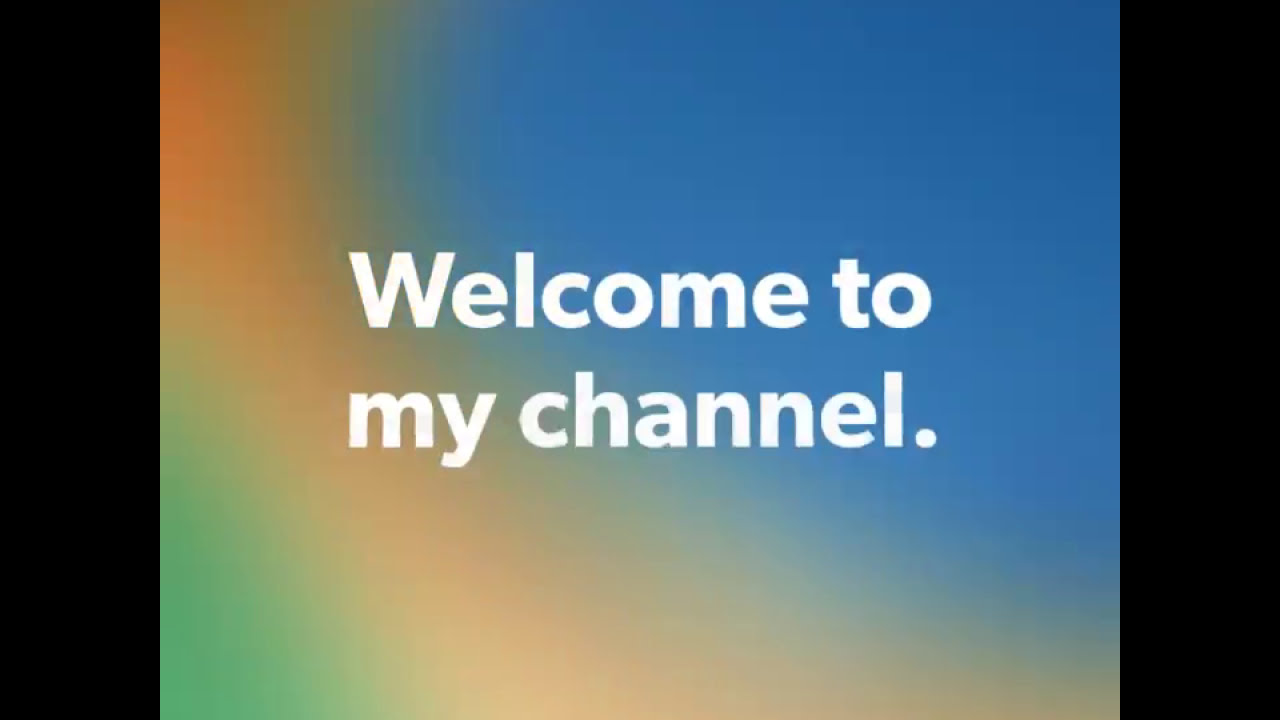The image features a vibrant, watercolor-like background framed by two vertical black stripes on either side. In the center, large white text reads, "Welcome to my channel" followed by a period. The background exhibits a smooth ombre effect starting with a small green triangle in the lower left corner, blending into light orange, then dark orange as it swishes from the top left towards the center. This transitions into a sky blue that dominates most of the background, flaring from the top right and encompassing the majority of the space down to the lower left, ending with a light green hue. The overall composition gives a dynamic and colorful introduction to the channel.